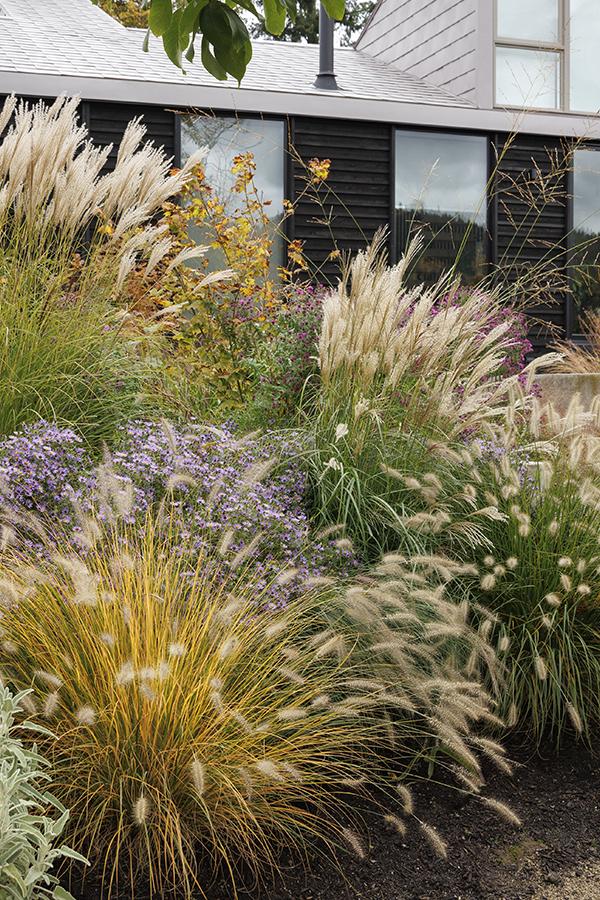The image captures a beautifully landscaped garden area in front of a well-maintained house with dark siding and a light gray roof. The house, partially obscured by the lush greenery, features several visible windows and a green tube extending from the roof. Dominating the foreground are expansive bushes of bunny tail grass and pampas grass, with their stems adorned in yellows, greens, and whites, capped with large, feathery, white plumes. Nestled among these grasses is a bush with tiny lilac flowers, possibly lavender, adding subtle hints of purple to the garden's color palette. Additionally, there is a bush with vibrant yellow flowers closer to the house. The overall arrangement of the garden is deliberate and well-designed, creating a serene and picturesque setting on what appears to be a beautiful day.